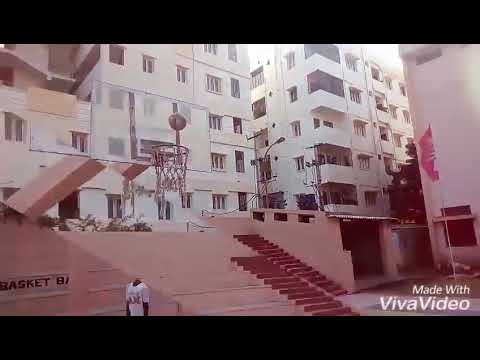The image features a large, somewhat blurry white apartment complex with multiple buildings consisting of five stories in height, showcasing both open and closed windows as well as balconies. Prominently in the foreground, there are red stairs and potentially a brown ramp leading up to the buildings. A disproportionately large basketball hoop with a ball going into it is superimposed in the scene, lacking a visible pole. At the bottom left of the image, a person wearing a white t-shirt with unreadable text is seen, but their head is cut off or obscured from view. The bottom-right corner displays the text, "Made with Viva Video," and just above it to the left, the partial word "basket" followed by a capital 'B' can be seen. Most of the bottom portion of the image has a pinkish hue contrasted with the red stairs, while the upper part features the white apartment buildings.